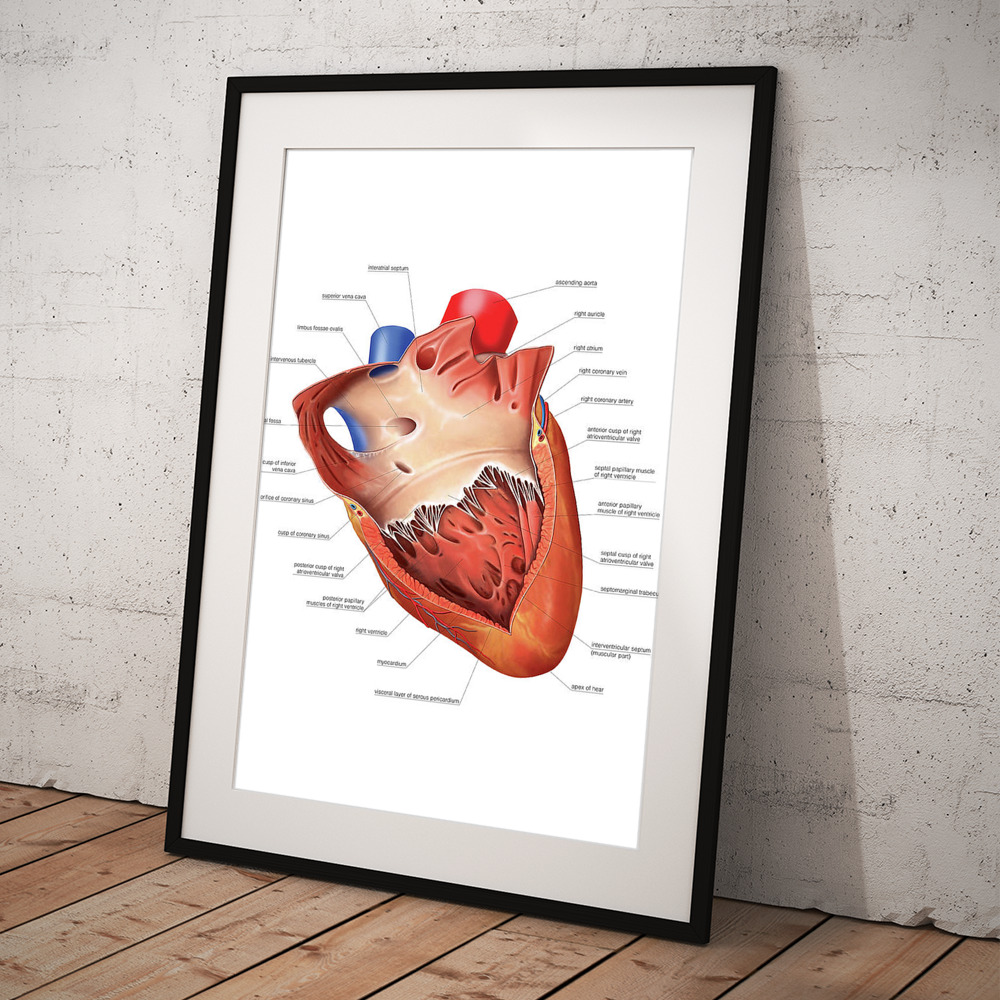The image showcases a detailed and vividly colored anatomical diagram of a heart, highlighting primarily the heart muscle in the center with an animated aesthetic. The heart is depicted in shades of red and orange, accented by blue pipes in the background, which likely represent major blood vessels. Inside the muscle, lighter white muscle fibers are also visible. Numerous annotations, written in black text, point to various parts of the heart, including terms like "ascending aorta," "right coronary vein," "right coronary artery," and "right ventricle," although the small text makes them somewhat hard to decipher. The illustration is framed within a border that features an inner tan band and an outer black wooden frame. It is set against a wooden floor, with a backdrop of a light gray stone wall. This image appears to be intended as an educational tool to highlight and teach different aspects of heart anatomy.